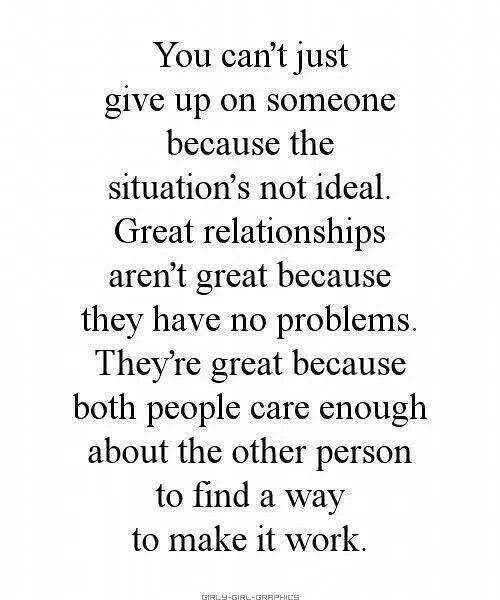The image features an inspirational quote presented in black text on a white background, arranged in a centered, typewriter-style serif font. The quote reads: "You can't just give up on someone because the situation's not ideal. Great relationships aren't great because they have no problems. They're great because both people care enough about the other person to find a way to make it work." The text spans twelve lines, with each line carefully centered and ample spacing between them. At the bottom of the text, there is a small, illegible credit. The composition is simple and clean, focusing entirely on the motivational message without any additional images, borders, or embellishments. The whole layout is in portrait orientation.